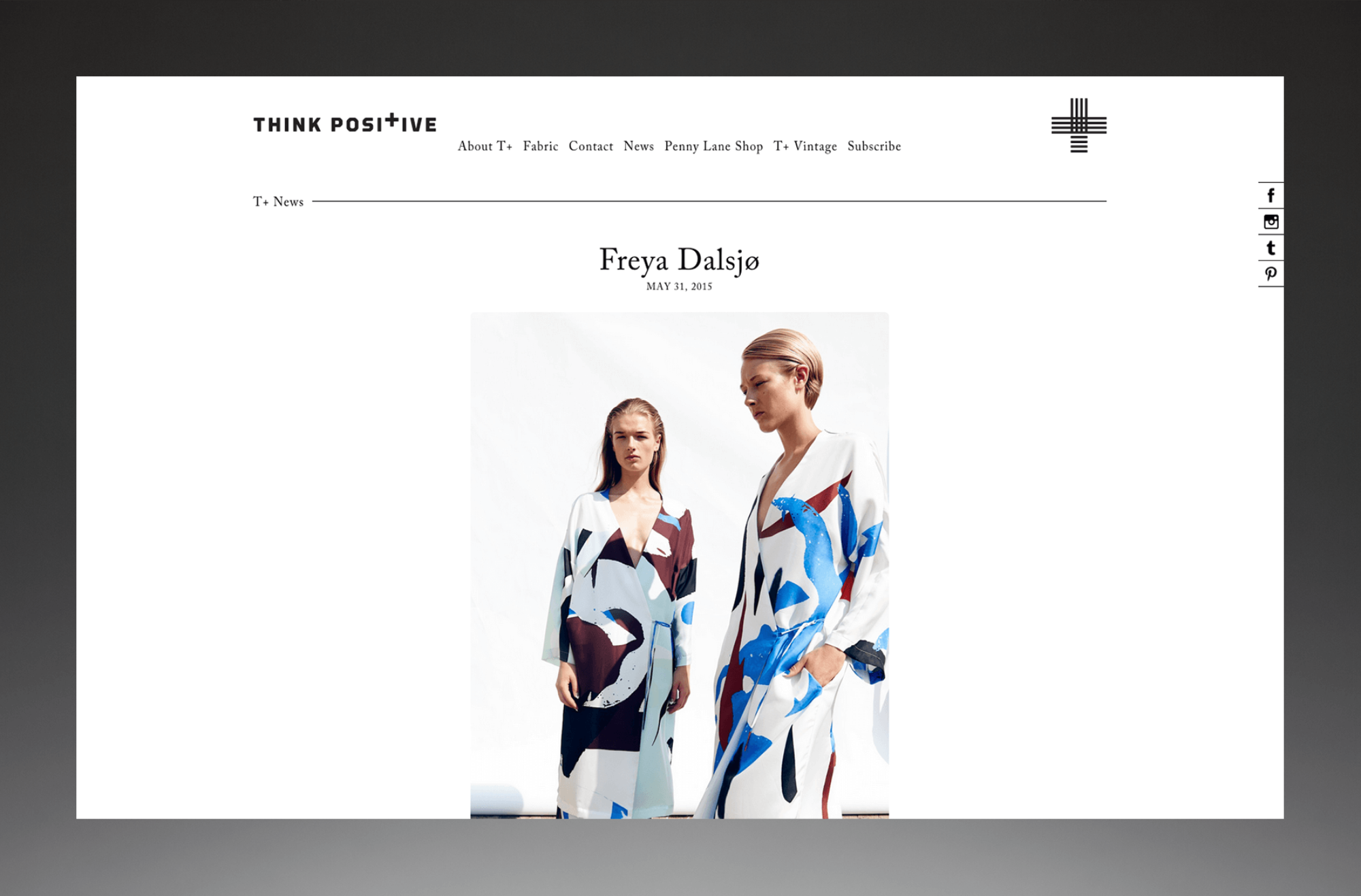This is a detailed description and cleaned-up caption for the image of the web page from the site "Think Positive":

---

The web page for "Think Positive" is elegantly framed, with the boundary resembling a sophisticated picture frame. The frame features a black tone at the top and along the sides, which gradually transitions into a lighter gray towards the bottom. The inner boundary of the frame is a soft gray, lighter in the center, creating a sleek and modern visual appeal.

Within this frame, the background of the web page is a clean, crisp white. Prominently displayed at the top are the words "Think Positive" in bold, black uppercase letters. Notably, the ‘T’ in “Positive” is cleverly stylized as a plus sign, adding a unique touch to the header.

Beneath the title, there is a navigation menu listing the available sections of the site. These include “About T Plus,” “Fabric,” “Contact,” “News,” “Penny Lane Shop,” “T Plus Vintage,” and “Subscribe.” This menu is elegantly presented in a smaller font than the main title, ensuring clarity and ease of navigation.

Dominating the main content area of the page is a striking photograph of two women modeling unique dresses. The first woman has her hair pulled back, which falls just below shoulder length, framing her face beautifully. The second woman sports a chic short bob haircut and is positioned side-on, adding dynamic angles to the photograph.

Both women are adorned in dresses featuring a white background with an array of abstract shapes in brown, blue, and black hues. These dresses are distinctive and draw the viewer’s attention, effectively showcasing the fashion offerings from "Think Positive".

---